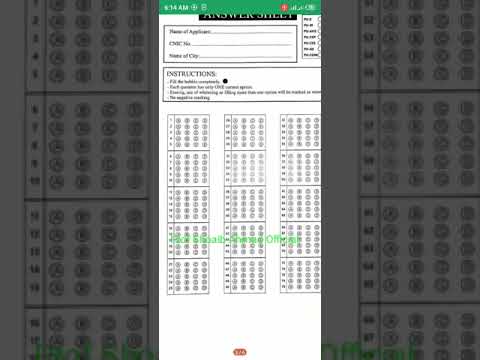The image is a color cell phone screenshot of an answer sheet, presented in portrait orientation, superimposed against a darker, landscape-oriented, enlarged version of the same image. The top part of the cell phone screen displays a green banner with the time "8:14 AM" and the battery life to the right. Below this is a dark banner, partially cropped off, with the title "Answer Sheet."

Beneath the title, there is a text box to enter the "Name of Applicant," an identification number, and city information, accompanied by bubbles designated for filling out responses. Following this box, a section titled "Instructions" is present, containing four bullet points. Below the instructions, the answer sheet is divided into three columns, each consisting of rows to fill in with a pen. Every row includes four bubbles labeled 'A,' 'B,' 'C,' and 'D,' none of which are filled in.

To the left and right of the central answer sheet, there are gray-toned, up-close sections of the Scantron form showing detailed bubble blocks labeled 'A,' 'B,' 'C,' and 'D' from top to bottom. The main image also displays some light green text or overlay about two-thirds down, and a red page number is visible at the bottom. The photograph is taken in a modern, photographic representational style.